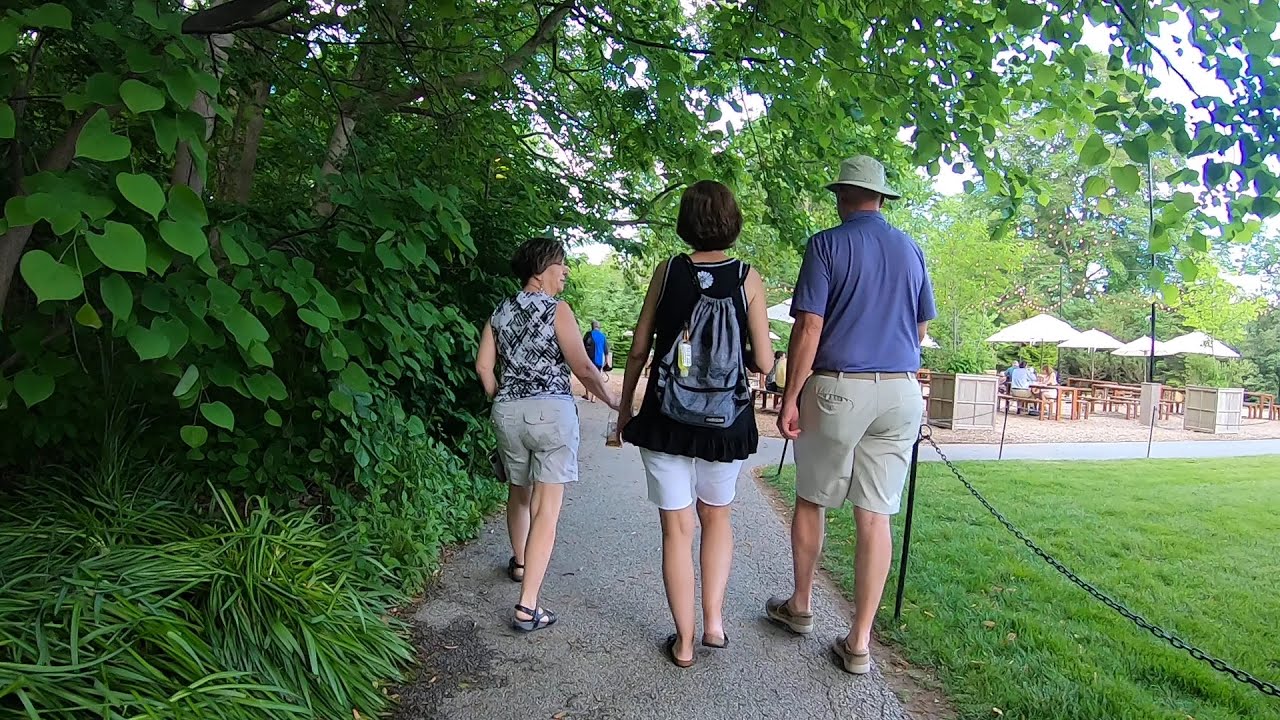This is an outdoor scene showcasing a calm, scenic landscape. The focal point is a group of three people walking along a roughly four-foot-wide asphalt trail, bordered by dense shrubbery, trees, and overgrown bushes on the left. The right side of the trail is defined by a grassy area, cordoned off with a metal chain to prevent entry. This grassy expanse features a seating area with picnic tables, each adorned with sunshade parasols, alongside wooden bins and trash cans.

Among the walkers, the man in the foreground is the tallest, dressed in tan khaki shorts, a light purple shirt, and tan tennis shoes. He also sports a khaki bucket hat. Flanking him, the women each wear light-colored shorts and sandals. The woman on the left wears a spotted white and dark brown tank top, while the woman in the middle has a black tank top and white shorts. In the background, another man in a blue shirt can be seen, likely adding depth to the tranquil park or arboretum-like setting.

The environment's predominant colors include lush green from the grass and foliage, with accents of white, purple, and black discernible in the walkers' attire. While a bit of the sky is visible, it's unclear whether it's partly cloudy. Notably, there are no animals in the scene.